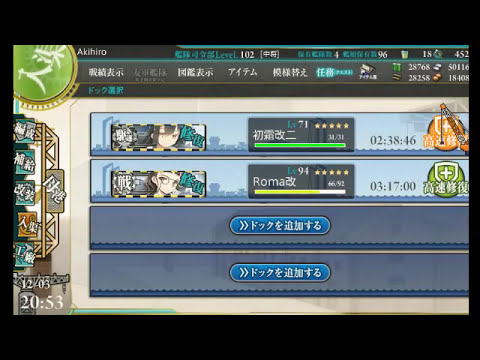The image is a screenshot from a video game, displayed in a landscape orientation with a black border. The screen is divided into multiple sections featuring various elements in Japanese and Chinese. At the top, there are four different banner bars, two of which show some kind of quest timer or match indicator, while the other two are blank, suggesting open slots for players or quests. 

In the top left corner, there's a green circle with Chinese symbols in white. On the left side of the screen, several Chinese characters are visible, hinting at the game’s instructions or dialogues. The central panel features two horizontal banners, each with manga-style illustrations of two girls accompanied by Chinese text, implying they are saying something. The names "Akihiro" and "Roma" and their levels or scores are displayed in a gray panel with white lettering in a mix of Chinese and Japanese.

To the right of the character illustrations, an orange circle with a white cross, partially covered by a crane image, and a green circle with a white shield and cross are visible. Additionally, blue ovals with white Chinese symbols lie beneath these elements. The lower left corner shows the date "1203" and the time "2053."

Overall, the image is detailed with an anime-inspired design, featuring intricate iconography that includes an orange pear-shaped circle, and a blue, green, and white color palette that emphasizes the game's navigational and status information.